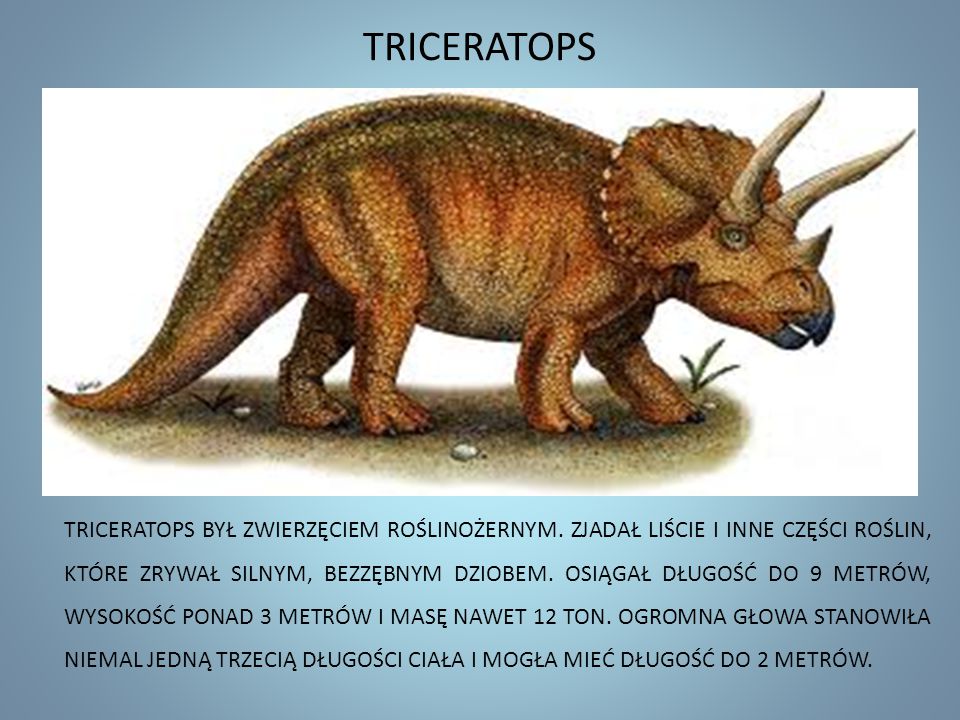The image is an artistic rendition of a Triceratops dinosaur characterized by its vibrant, earthy color palette, predominantly featuring red, brown, and dark beige hues. The Triceratops, depicted with two large horns protruding from its head and a horned nose, is shown walking on four sturdy legs on a simple, stony ground with a small plant emerging on the right side. The background is mostly white with a light blue outline around the edges, directing focus onto the dinosaur positioned centrally but slightly towards the top. Above the dinosaur, the title "Triceratops" is prominently displayed in all capital letters in black font. Below the Triceratops, there are four lines of black text in Polish, providing additional context or description. This detailed and vivid presentation, reminiscent of an educational PowerPoint slide, suggests the image may be used for informative purposes.